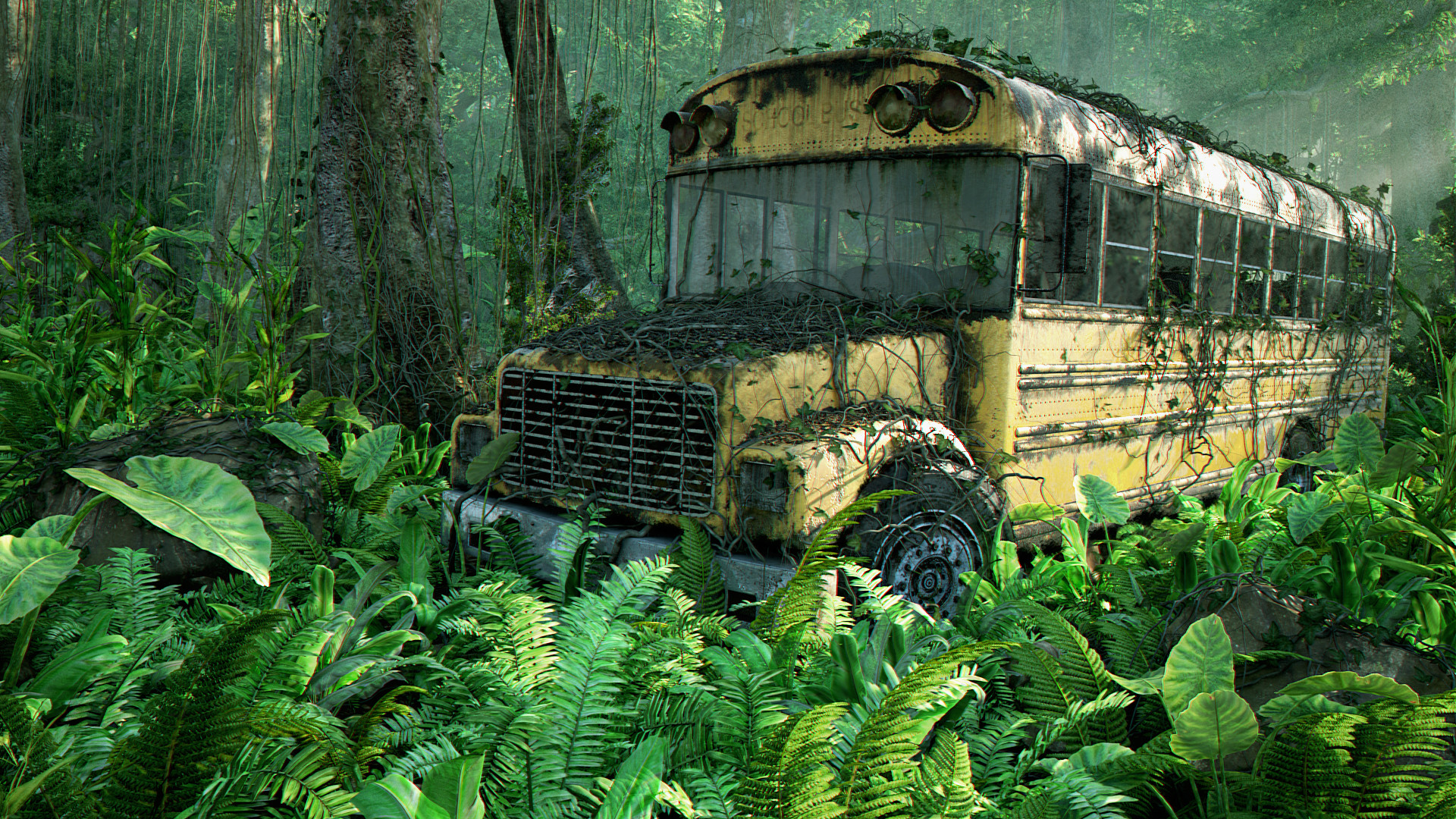The image depicts a realistic, dystopian scene set within a dense, overgrown rainforest. Dominating the right side of the frame is an old, rusted yellow school bus, with faded "school bus" lettering and broken windows, that looks like it has been abandoned for a significant amount of time. The bus is enveloped in lush greenery, with plants, branches, and vines overtaking its structure—climbing up its sides, spilling over its roof, and even growing out from within. The tires are weathered, and the front lights are rusty. Thick trees surround the bus, their canopies so dense that no sky is visible, plunging the scene into a twilight of greens, blacks, and yellows. Near the bus's front, scattered vegetation and rocks punctuate the forest floor, adding to the sense of long-standing abandonment in this heavily vegetated area. The tableau suggests a world reclaimed by nature, with the eerie ambiance of a forgotten past.